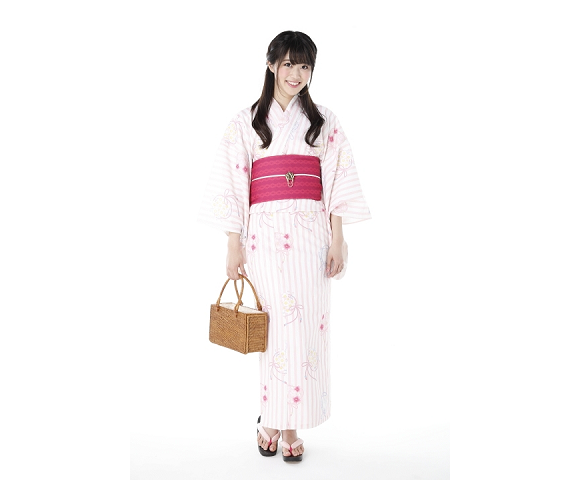This full-body photograph features a young Asian woman dressed in traditional attire. Her long brown hair, pulled back at the sides with two wisps framing her face, cascades down past her shoulders. She is smiling and looking directly at the camera. The outfit is a form-fitting, floor-length dress adorned with pink and white stripes, complemented by scattered cherry blossoms. The dress has quarter-length sleeves and is cinched at the waist with a thick pink belt. She is carrying a wicker handbag in her left hand and wearing pink sandal-like shoes with a pink toe piece and black bottoms. The background of the image is completely white.